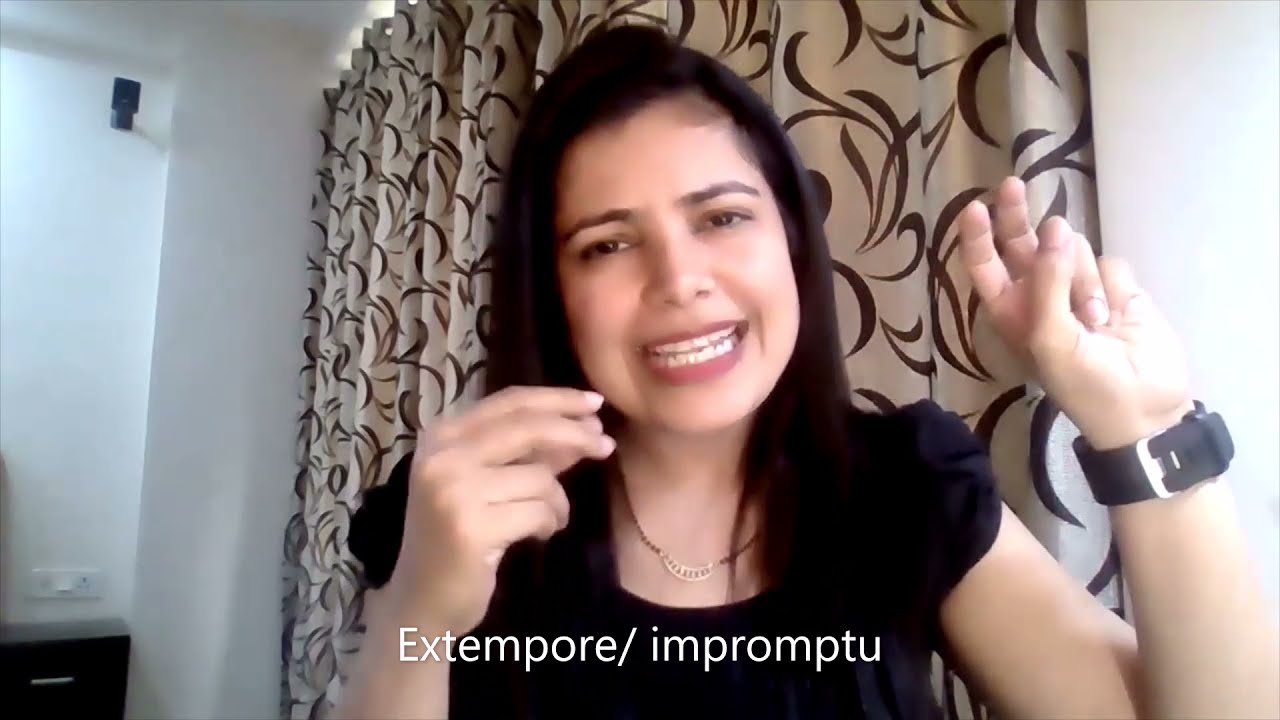The photo captures a young woman, likely in her late teens to early twenties, standing at the center. She is set against a white curtain adorned with black or brown swirls, which resembles a shower curtain, suggesting she might be in a bathroom or similarly styled room with white walls. Behind her, a hallway or vanity is faintly visible. 

Her dark hair is pulled back from her forehead with soft strands falling around her neck and over her shoulders. She has dark eyebrows, twinkling eyes, and her expression conveys mixed emotions—it’s a blend of happiness, indicated by her wide smile with slightly parted lips, and a hint of distress. She wears a black, short-sleeved top with a scooped neckline, and a gold necklace around her neck.

Her left arm is bent at the elbow with her hand just in front of her face, her thumb and pinky touching while her index and middle fingers are partly extended. Her right arm, also bent at the elbow, holds her hand up near her shoulder, possibly capturing a finger-snapping motion. A wide watch band is visible on her right wrist. Text at the bottom of the photograph reads, "EXTEMPORE / IMPROMPTU."